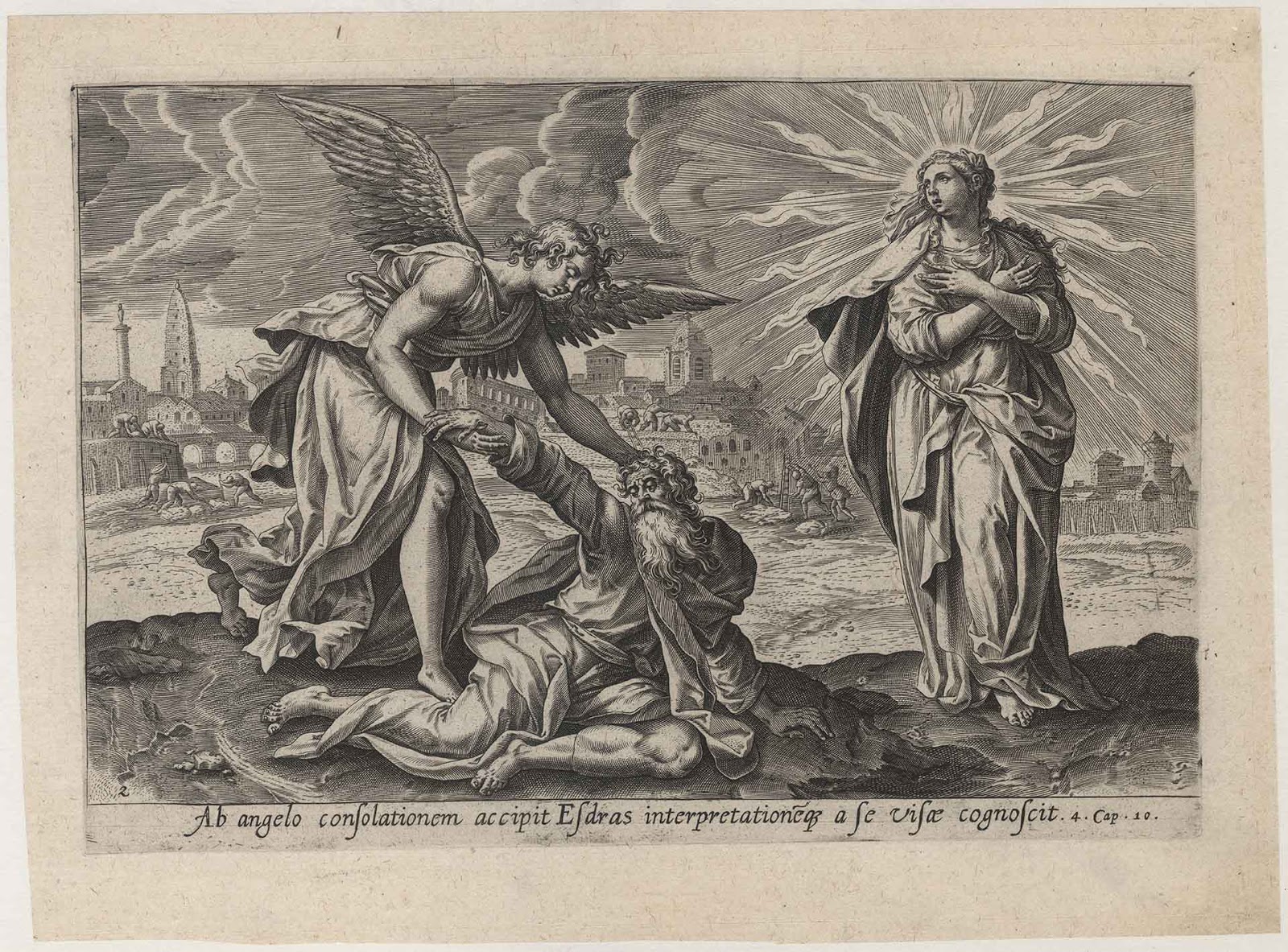The image is a detailed, classical black-and-white engraving, possibly from the 16th or 17th century, rendered on beige-colored paper. It depicts a poignant, biblical scene with three central figures set against the backdrop of an ancient cityscape. On the right, a radiant woman dressed in flowing robes stands with her arms crossed over her chest, her head adorned with a halo-like aura of flames. To her left, an angel with two wings bends down toward an elderly man with a long white beard, who is either fatally wounded or deceased. The angel gently cradles the man's head with one hand while holding his hand with the other, suggesting a moment of divine assistance or passage. The trio is positioned on a hill overlooking the distant city, with clouds and a shining sun visible in the sky above. Beneath the scene, there's a phrase written in Latin, adding an ancient and sacred touch to the artwork.